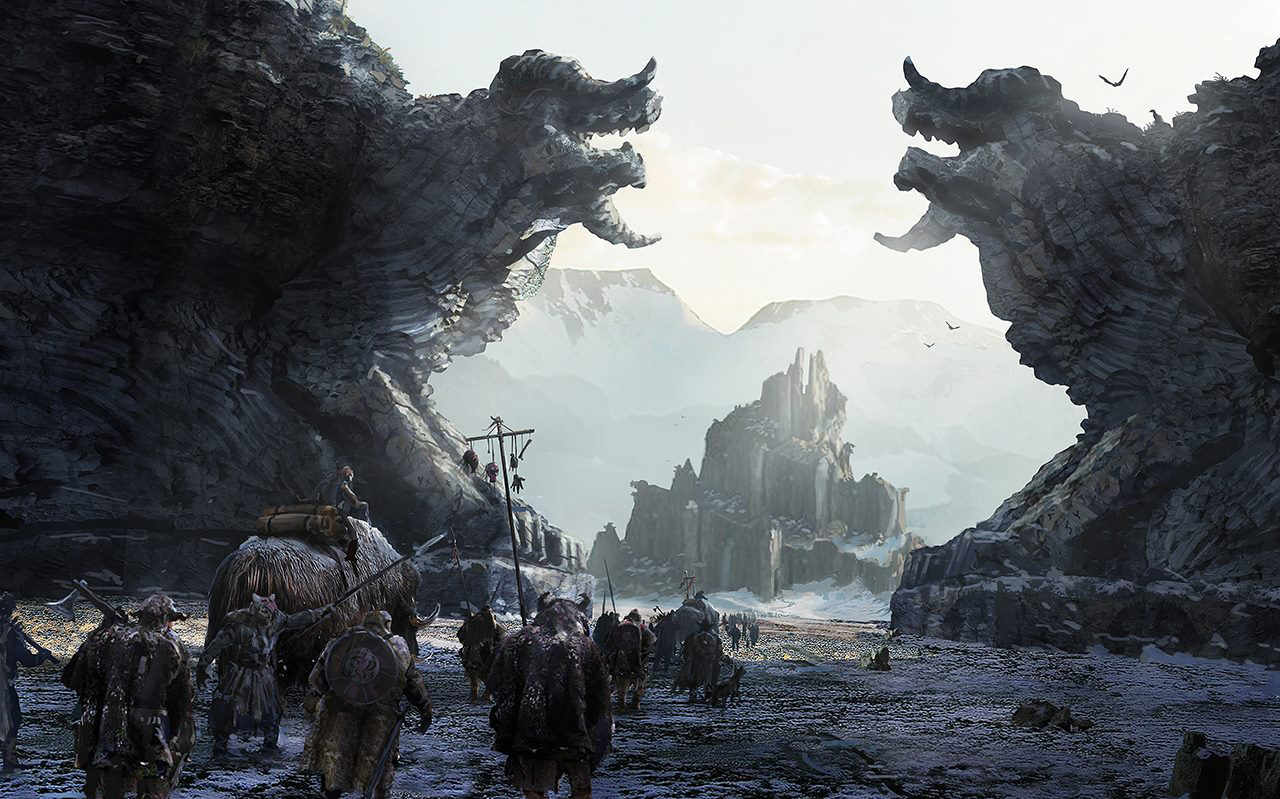This intricate painting, featured in the illustrated book "Fall of Gods" by Rasmus Berggruen, captures an ancient and fantastical outdoor setting reminiscent of medieval or Viking times. The scene shows a procession of dozens of individuals clad in animal skin garb, horned helmets, and ancient attire suited for cold weather. They march in a column from the left foreground, through a narrow valley formed by two colossal hills, and extend into the background. Each hill is adorned with elaborate, dark bluish-gray stone carvings resembling mythical creatures with tentacled heads, ominously framing the pathway.

In this atmospheric landscape, the group carries shields, spears, axes, and a tall cross adorned with dangling artifacts, evoking a sense of a crusade. One notable figure is riding a large, fantastical beast—a hybrid between a buffalo and an elephant, complete with tusks and horns. Above the marching column, ancient birds soar under an overcast sky, adding to the mystique.

The end of their path reveals a sunlit spiral castle, behind which majestic snow-covered mountains rise. This imposing structure, possibly an eroded volcano cone, serves as their destination. This detailed and immersive tableau seamlessly blends elements of myth, history, and fantasy, offering viewers a narrative steeped in ancient legend.